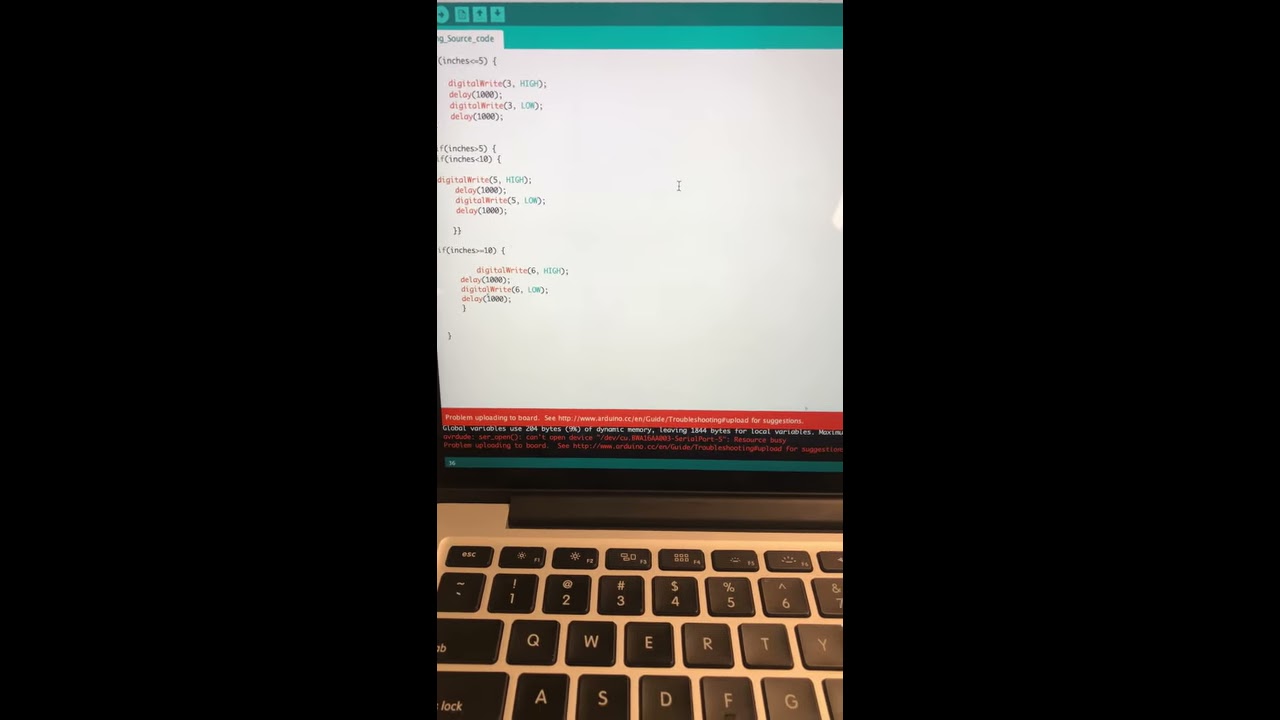The image is an indoor setting with a dimly lit environment, captured in a detailed photographic style. At the forefront of the photo is a white or gray laptop keyboard with black keys, showing recognizable keys such as the 1 through 6 digits, the QWERTY row, as well as the tab, escape, and back buttons. Centered on the screen is a detailed view of a code editor featuring a series of code prompts, numbers, and parentheses in various colors. The main coding area on the screen is white with small, intricate, and difficult-to-read text in red, green, and black fonts. The screen is framed by a bluish-green top border and a red footer at the bottom. Additionally, the left and right panels of the image are black, highlighting the central panel displaying the coding interface. There are no people visible in the photograph.